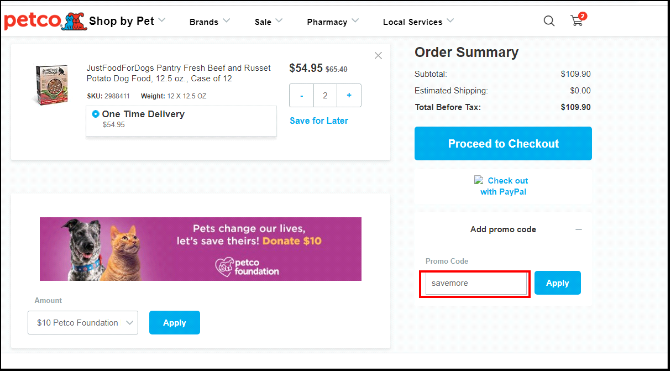This screenshot captures a detailed view of the Petco website. In the upper left-hand corner, the iconic Petco logo in blue and red is prominently displayed. Adjacent to the logo in the header section are several dropdown menus labeled "Shop by Pet," "Brands," "Sale," "Pharmacy," and "Local Services." Moving further right, there is a search icon followed by a shopping cart icon, which displays a small circle with the number "2," indicating two items are in the cart.

Directly beneath this header, an "Order Summary" section provides a detailed breakdown of the shopping totals, including the subtotal, estimated shipping, and total before tax. Below this section is a large blue button with white text that reads "Proceed to Checkout." Additionally, there is an option to "Checkout with PayPal," represented with a broken image link, and an area to add a promo code. Within this section, a highlighted red outline surrounds the input box, which contains the text "save more," accompanied by a blue "Apply" button.

Shifting to the left side of the screen, the shopping cart contents are displayed. The main item is "Just Food for Dogs Pantry Fresh Beef & Russet Potato Dog Food" priced at $54.95 each, with a quantity of two. The shipping method is specified as "One-time Delivery." Directly below this, an advertisement with a purple background captures attention. The ad features a message, "Pets Change Our Lives," and encourages donations with the text "Donate $10 to Petco Foundation." To the left of this text, there are two pets: a dog with black and gray fur and a beige-furred cat. The donation section includes an "Amount" label, specifying "$10 Petco Foundation," and a blue "Apply" button with white text.

This comprehensive description effectively outlines the visual elements and information conveyed in the Petco website screenshot.